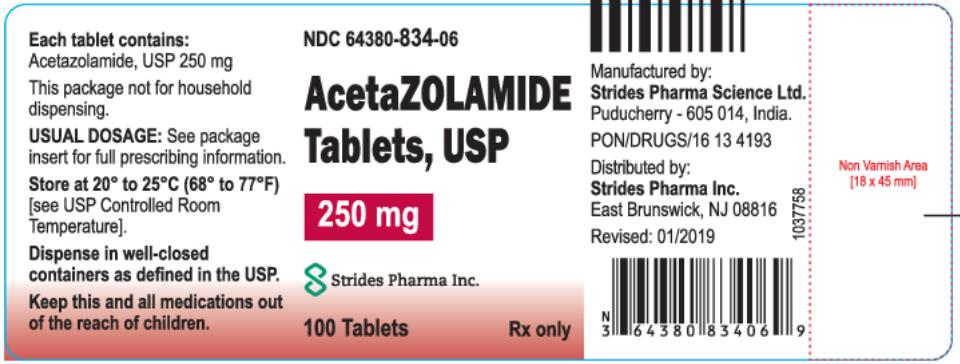**Descriptive Caption for Medication Label Image:**

The image showcases a detailed medication label for Acetazolamide tablets, USP 250 mg, designed prominently with essential prescribing and storage information. 

**Left Section:**
- Each tablet contains acetazolamide, USP 250 mg.
- Statement: "This package not for household dispensing."
- Usage Instructions: "Usual doses" (highlighted in bold).
- Reference: "See package insert for full prescribing information."
- Storage Conditions: "Store at 68 to 77°F (see USP controlled room temperature)."
- Dispensation: "Dispense in well-closed containers as defined in the USP."
- Safety Warning: "Keep this and all medications out of the reach of children."

**Center Section:**
- NDC number: "NDC 64380-83406" at the top.
- Medication Name: "Acetazolamide Tablets, USP" in large print.
- Strength: "250 mg" just beneath the medication name.
- Company Logo: A green logo labeled "Strides Pharma Incorporated."
- Quantity and Usage: "100 Tablets" and "For prescription use only" at the bottom.

**Right Section:**
- Barcode Presence.
- Manufacturing Information: "Manufactured by Strides Pharma Science Ltd, Puducherry 605014, India."
- Identification Code: "PON-DRUGS-1613-4193" in all caps.
- Distribution Details: "Distributed by Strides Pharma Inc., East Brunswick, New Jersey 08816."
- Revision Date: "Revised 1-2019."
- Additional UPC Code: Present with an adjacent non-varnish area (18x45).

The label includes a designated white space marked next to a red dotted line, indicating a "non-varnish area."